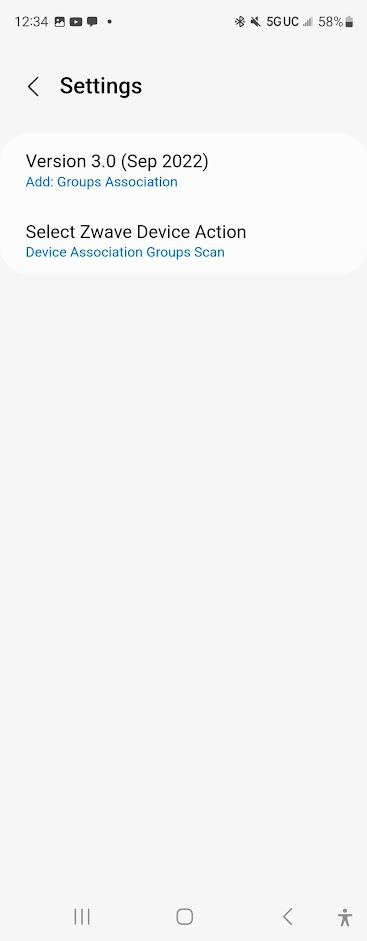In this detailed screenshot of an Android device, the top-left corner displays the current time as 12:34. The device shows several app icons including Gallery, YouTube, and Messages. Additionally, the Bluetooth icon indicates an active connection to either headphones or a speaker, and the device is set to mute. The 5G connectivity is strong with 4 out of 5 bars, while the battery status is at 58%.

The interface shows text pertaining to "Settings," marked as version 3.0, dated September 2022. There are various options listed such as "Add," "Groups," "Association," "Select with Device," "Action," and "Scan." Below this section, the navigation bar features buttons for recent apps, the home screen, and debugging functions. The overall layout and features confirm this as an Android device.